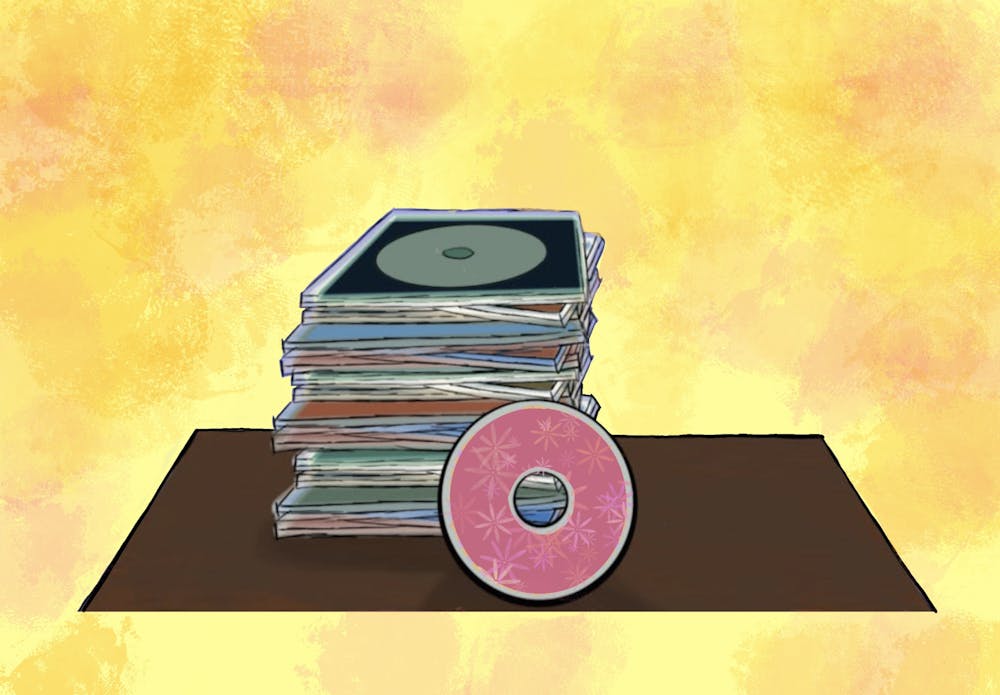This is a cartoon illustration of a stack of CDs placed on a brown desk or bureau, featuring a textured background with a mix of orange, yellow, peach, and pink hues, creating a sponged appearance. The stack of CDs, numbering between 15 and 20, is housed in plastic cases and arranged haphazardly, with some cases poking out at various angles. In front of this uneven pile rests a distinctive pink CD adorned with floral and star-like patterns in lighter pink or white, and a black-shaded outer rim. The overall composition is bright and visually engaging, with the chaotic stack contrasting against the vibrant backdrop.